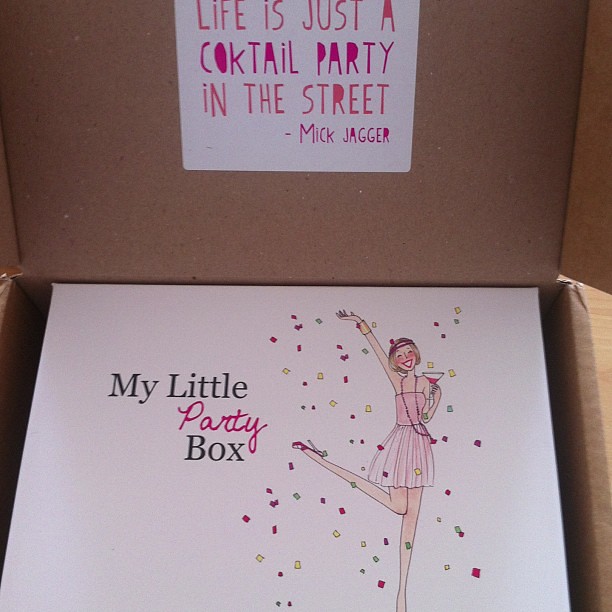An open cardboard box with its lid flipped up reveals a festive scene. The inside of the lid features a light pink paper with a handwritten quote in orange and purple lettering that reads "Life is just a cocktail party in the street – Mick Jagger." The word 'cocktail' is misspelled, missing the 'c' after the 'o.' Positioned in the bottom left corner of the box is a smaller white box labeled "my little party box," with the word "party" written in pink cursive. To the right of this smaller box, there is a drawing of a vibrant, thin woman dancing. She is wearing a strapless pink dress, adorned with a dark purple necklace that drapes down to her waist. Her blue hair is accented by a thin purple bandana, and her face is brightly animated with a big smile and red accents. The woman holds a cocktail in one hand while her other hand is raised high above her head. Her left leg is bent dramatically, extending behind her. Around her, square confetti in various colors—red, yellow, green—adds to the celebratory atmosphere.